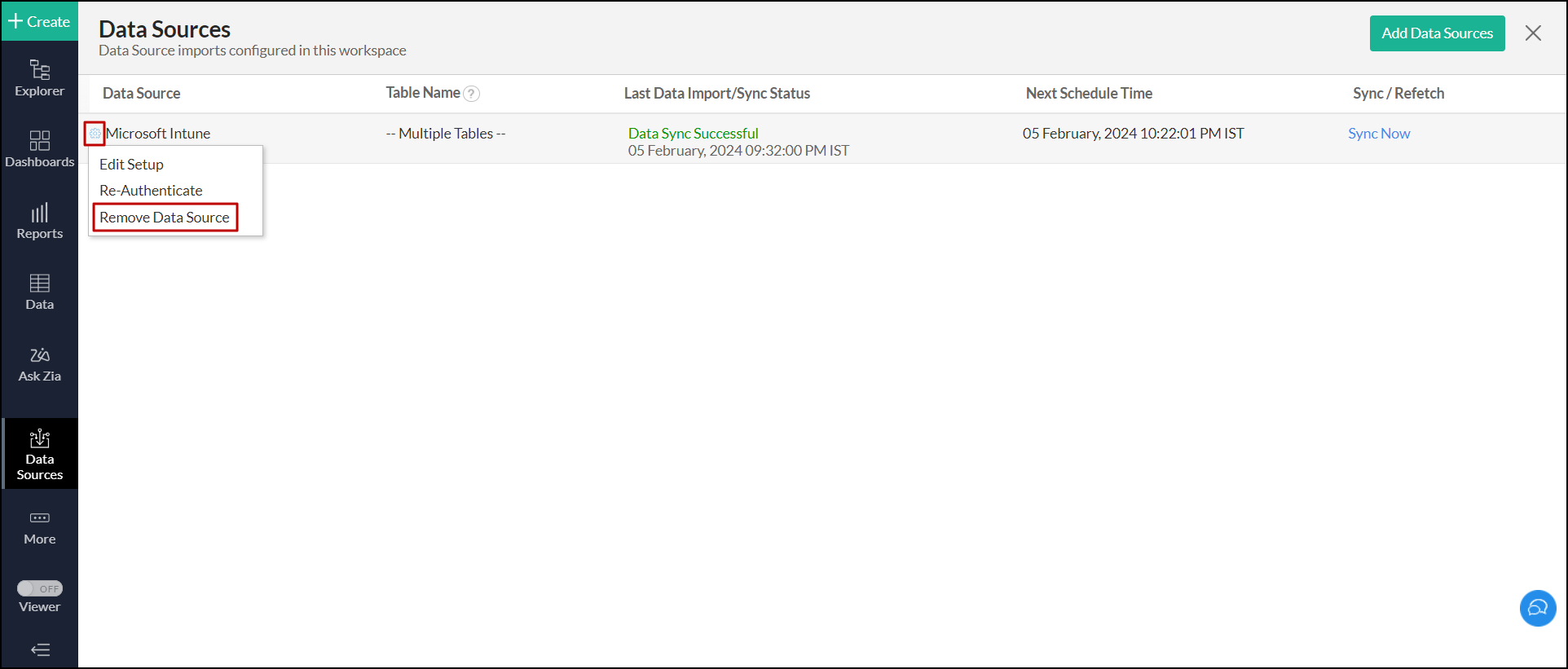This image showcases a web interface for managing data sources. The left-hand side features a black index panel with a series of labeled icons arranged vertically. At the top of this black panel, there is a gray rectangular button with a white plus sign and the word "Create" in white, oriented vertically. Below this button, the navigation panel includes the following labels, each accompanied by an icon: "Explorer," "Dashboard," "Reports," "Data," and a small, unreadable label suggestions followed by "Zia." Further down, there's another icon followed by the phrase "Data Sources" and an additional icon with the label "Views." At the very bottom, there are three horizontal lines indicating more options.

The main section of the page is predominantly white with a gray banner stretching across the top. On the left corner of this gray banner, bold text reads "Data Sources," while directly below it, smaller text states "Data Source Import Configuration in This Workspace." On the right side of the gray banner, there is a prominent green rectangular button labeled "Add Data Services."